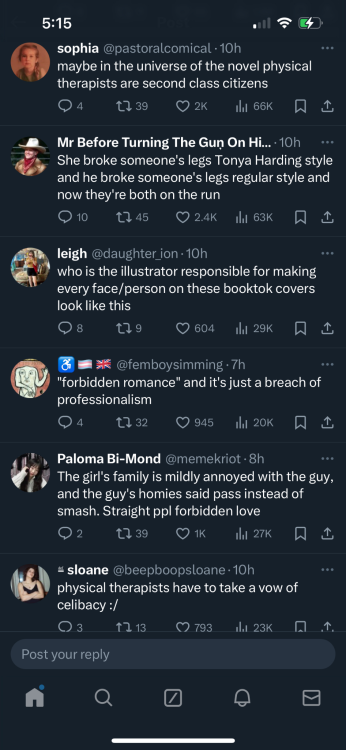A vertically-oriented image captured from a smartphone screen displays a Twitter feed against a dull black background. The top-left corner of the screen shows the time, "5:15," in white text, while the top-right corner features several icons: a signal bar strength indicator, a Wi-Fi icon, and a battery life indicator, which is green with a lightning bolt, indicating that it is charging.

The feed starts with a tweet from user Sophia, whose handle is @PastoralComical. Her profile picture is a circular image situated on the left. The tweet, posted "10 hours ago" in gray text, reads: "Maybe in the universe of the novel physical therapists are second-class citizens." Below this tweet, the icons for comments, retweets, likes, views, sharing, and bookmarking are visible.

The next tweet is by a user named Mr. before turning the gun on himself, posted "10 hours ago." The tweet states, "She broke someone's legs Tanya Harding style and he broke someone's legs regular style and now they're both on the run." Identical engagement options follow this tweet.

Following that, Lee, with the handle @DaughterIon and posting "10 hours ago," questions: "Who is the illustrator responsible for making every face/person on these book covers look like this?" 

Next, a user with a profile picture featuring multiple flags and the handle @FemboySimming, tweeted "seven hours ago": "'A forbidden romance' in quotations, and it's just a breach of professionalism." Engagement icons are also present below this tweet.

Subsequently, Paloma B Mon posted: "The girl's family is mildly annoyed with the guy and the guy's homie said pass instead of smash. Straight people forbidden love," followed by the standard engagement options.

Lastly, a user named Sloan with a profile picture tweeted: "Physical therapists have to take a vow of celibacy," accompanied by the same interactive icons as the previous posts.

At the bottom of the screen, the navigation bar includes icons for Home, Search, Notifications, and Direct Messages, representing various Twitter functions.